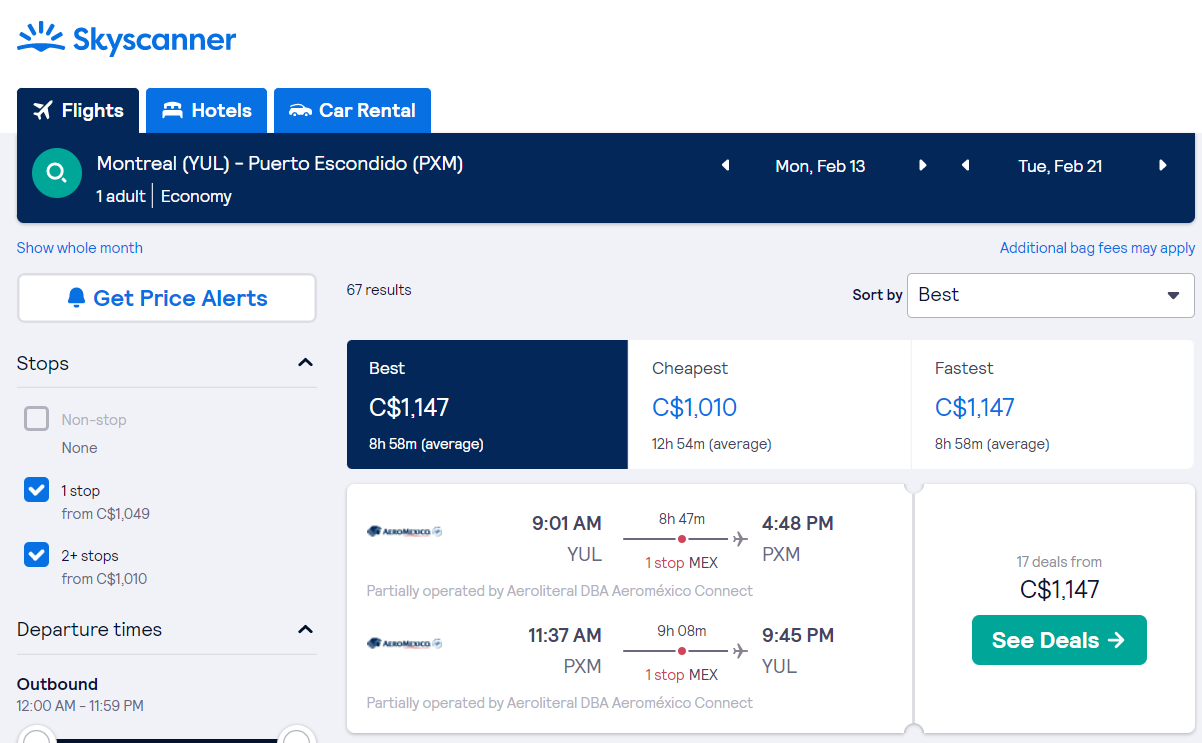This is a screenshot from Skyscanner's website depicting flight options for a trip from Montreal to Puerto Rico. The search parameters include one adult in economy class. The interface offers the ability to search for flights, hotels, and car rentals, all available via selectable tabs. Located in the top left corner, there is an option to "Get Price Alerts." The user can view flight prices for the entire month and has selected a search with one stop, as well as options for two or more stops starting from $1,010. The one-stop flight prices begin at $1,049, with listings sorted from the cheapest to the fastest flights. The "Best Price" option is highlighted at $1,147. The travel dates specified are from Monday, February 13th, to Tuesday, February 21st. In the top right corner, there is a drop-down menu labeled "Sort by Best," which organizes the flights by the best deals. Additionally, it shows that there are 17 offers starting from $1,147, also listing details for departure times and outbound flights.